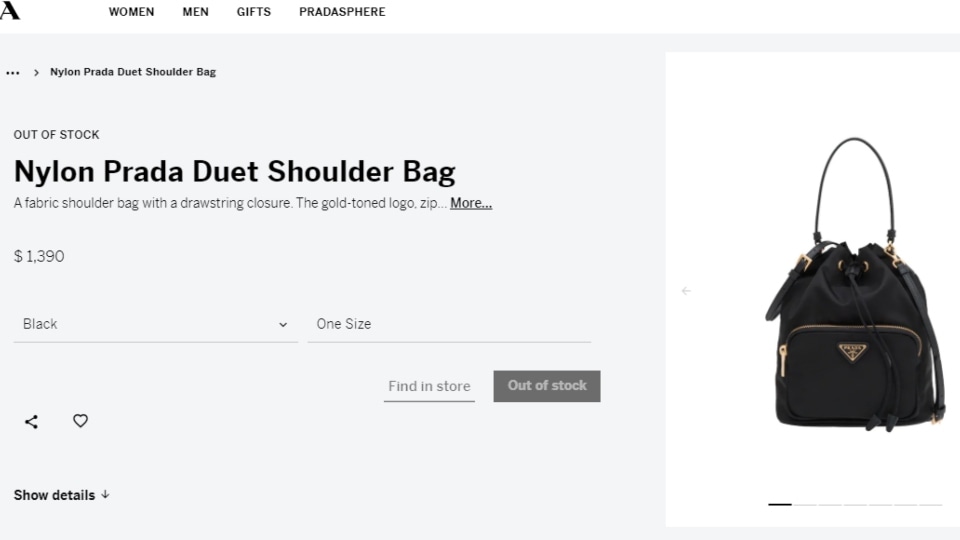Screenshot of a Prada Duet Nylon Shoulder Bag on an Online Retail Website

The screenshot features the interface of an online retail sales site, showcasing a Prada Duet Nylon Shoulder Bag. The top of the page has a clean, white header with a stylish "A" logo, followed by navigation links for various sections: Women, Men, Gifts, and Protosphere. Beneath the header, there's a light gray rectangular section containing the product details. The product is identified as "Out of Stock Nylon Prada Duet Shoulder Bag."

The description highlights that the bag is a fabric shoulder bag with a drawstring closure and features a gold-toned Prada logo. There’s additional information available through a "more" link. The bag is priced at $1,390. The color option visible is black, and beside it, there is a note saying "One Socks," likely indicating a related product or accessory.

Below this, there are two buttons: "Find in Store" and "Out of Stock." There are also icons for sharing the product and liking it, with a "Show Details" link in darker font for more thorough information on the bag.

On the right side of the screenshot is a detailed image of the product. The Prada Duet Nylon Shoulder Bag, shown in black, resembles a compact backpack with an extended handle. It features a front zipper compartment adorned with the iconic Prada logo.